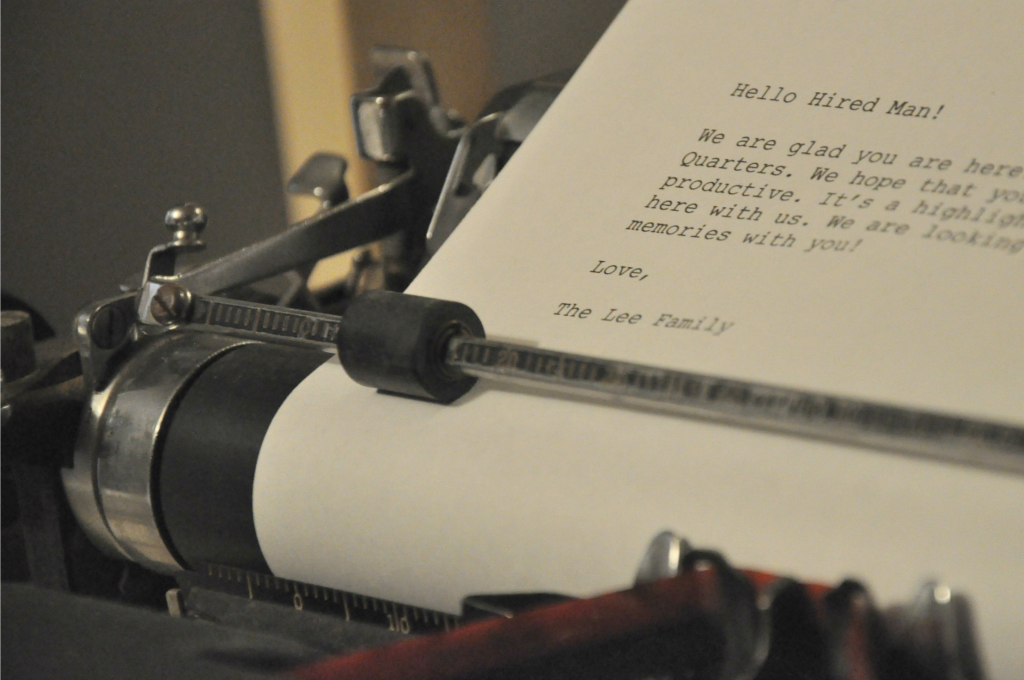This is a close-up photo of a black and silver typewriter, with the focus on the reel and the rubber roller wheel. The typewriter appears new and in good working condition, resting as if it has completed its task. A piece of white paper is inserted into the typewriter, slightly offset to the right, with typed text visible but partly cut off by the frame. The readable text says, "Hello, hired man. We are glad you are here. Quarters. We hope that you productive... here with us. We are looking... memories with you. Love, the Lee family." The background suggests the typewriter is in a room, with parts of a table leg and dark gray elements visible. The middle and bottom of the image show the bars that hold the paper, and there's a hint of a red ribbon towards the bottom center of the picture.